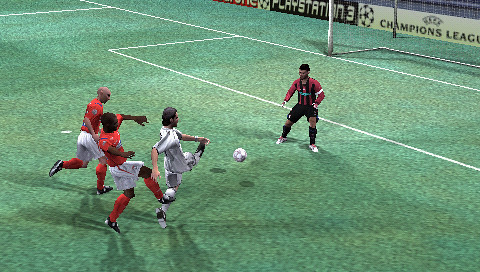In this freeze-frame from a soccer video game, a high-stakes moment unfolds on an artificial green playing field. A breakaway is in progress with a player in white, who has just released a kick towards the goal. The goalie, dressed in black shorts, black shin guards, white shoes, and a distinctive red shirt with a white stripe down his left sleeve, has come out of the box to reduce the angle. The goal's silver stanchions and parts of the net are visible, though the net itself is somewhat obscured.

In the background, advertisements for "PlayStation 3" and the "Champions League" are prominently displayed along the stadium wall, with the latter accompanied by a soccer ball icon. The stadium seating appears empty, revealing rows of silver chairs. Behind the white-clad player, two opponents in orange jerseys with white shorts and orange knee socks scramble to catch up, one seemingly too late to intercept as the ball hurtles towards the goal. The scene captures a moment brimming with tension and anticipation against the backdrop of a vividly-rendered virtual soccer arena.